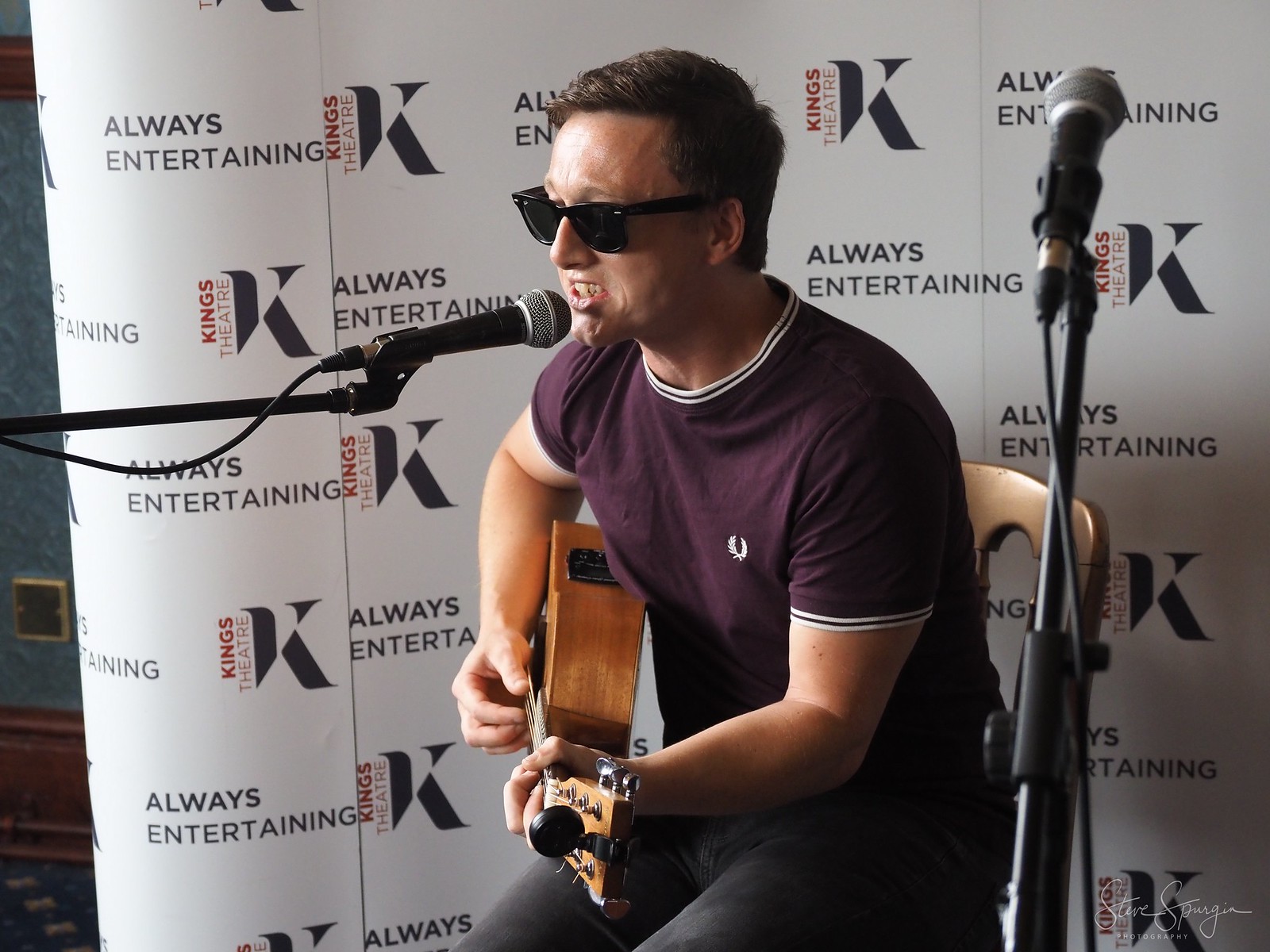A detailed photograph captures a Caucasian man with dark hair, wearing black sunglasses, sitting on a chair while passionately singing into a microphone. He is playing a wooden guitar and is attired in a short-sleeved, maroon (or dark mulberry colored) t-shirt with a white logo on the upper right side of the chest, along with dark pants. The microphone he sings into has a silver head and a black base, and another unused microphone can be seen on the right edge of the image. The man appears deeply absorbed in his music, looking slightly off to the left with his mouth open. Behind him, a white prop wall features a repeating pattern of the text "always entertaining" and "King's Theatre" with a prominent red K. The rest of the text is in black, and there is a blurred signature at the bottom, unreadable except for the name "Steve".